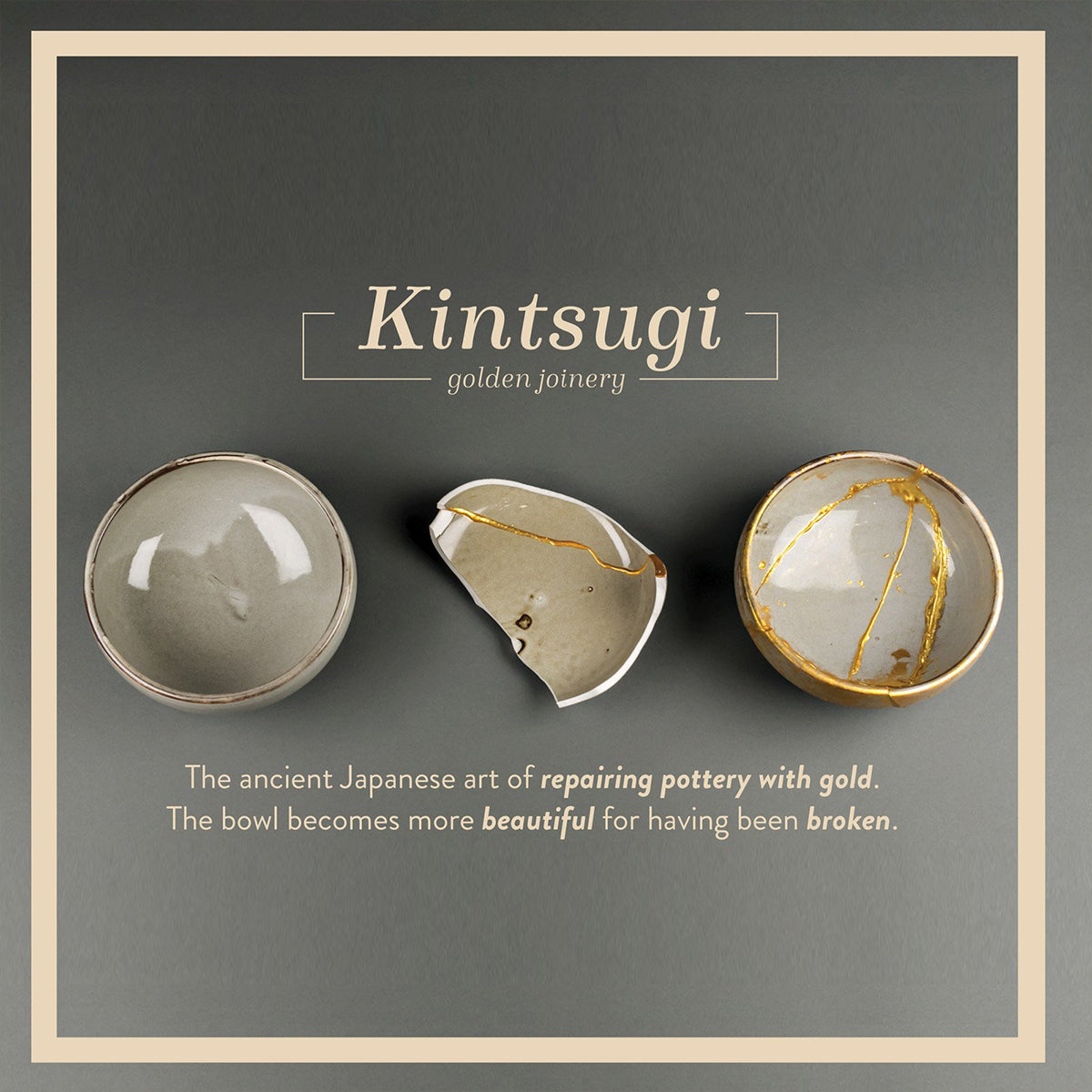The image is an advertisement or educational poster with a dark gray background that fades to a lighter gray towards the bottom, framed by a beige square border. In the center of the image are three ceramic bowls, all in a beige color with a polished finish. The bowl on the left is intact and plain. The middle bowl is broken and partially repaired using the kintsugi technique, where the cracks have been filled with gold pigment. The bowl on the right is fully restored with prominent gold-filled cracks. At the top of the image, the word "kintsugi" is written in a special font, with "golden joinery" below it in smaller letters. At the bottom of the image, descriptive text reads, "The ancient Japanese art of repairing pottery with gold. The bowl becomes more beautiful for having been broken," emphasizing the cultural and aesthetic significance of the practice. The glossy finish of the ceramics reflects studio lights, adding a shiny, polished look to the overall composition.